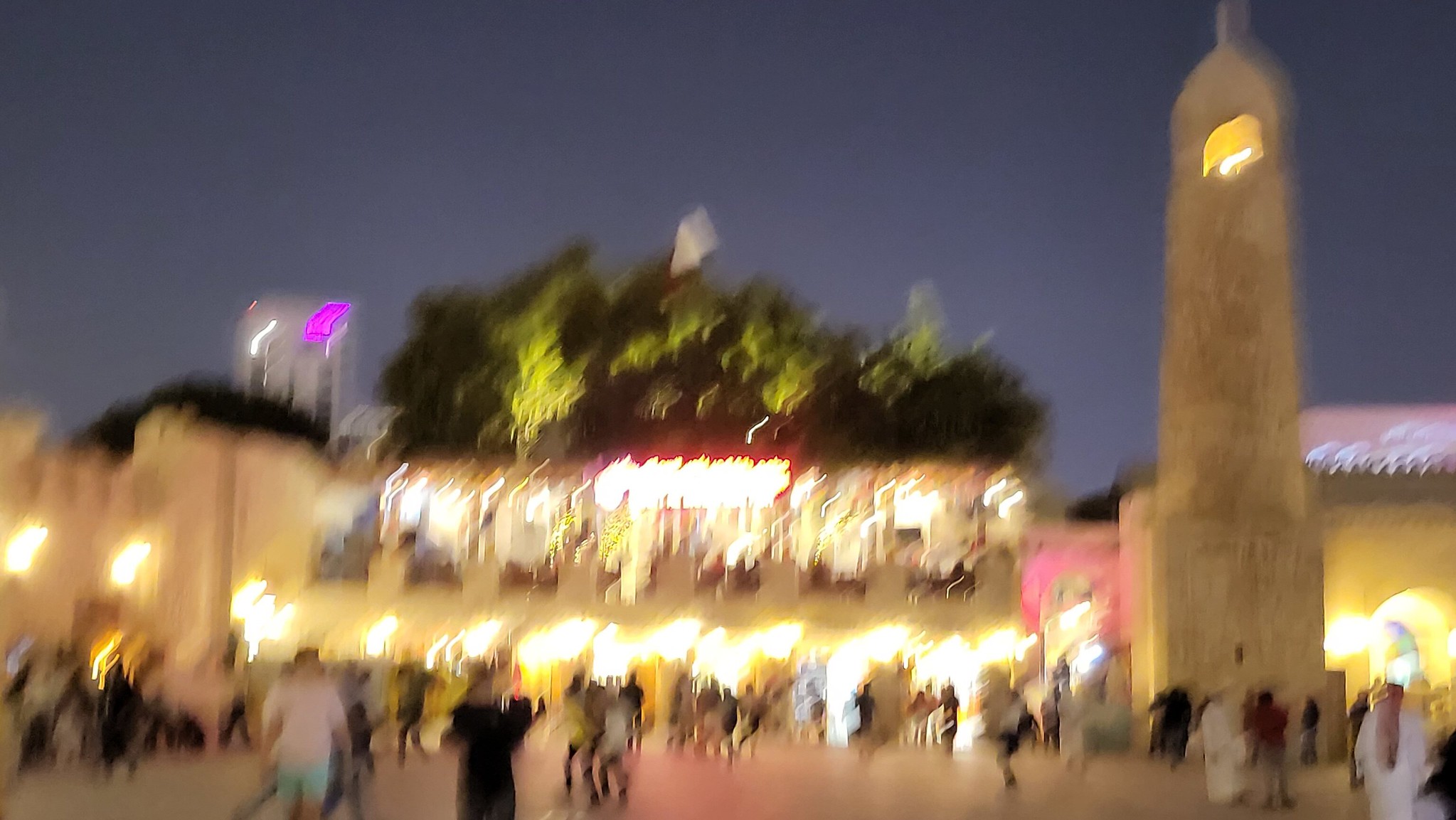This is a very blurry nighttime image of a bustling outdoor shopping and entertainment area, resembling a market square with vibrant activity. Central to the scene is a large, metal pillar with a light at the top, featuring a rounded upper section and a square stone base. The background reveals a two-level, well-lit building, adorned with lights both at the top and bottom. The upper level appears to host a dining area with people on the balcony, while the lower level teems with people walking. A red neon sign is faintly visible on the upper level of the central building. To the right, an arched walkway or pass-through doorway is apparent, contributing to the castle-like architecture of the area. Above the building, the tops of a few illuminated green trees are visible, along with a tall building in the distance towards the left. The scene also includes a noticeable clock to the right and numerous people dressed in varying styles, indicating perhaps a warm evening. The overall ambiance is lit by many bright lights, suggestive of a lively dining or shopping plaza surrounded by stone structures.